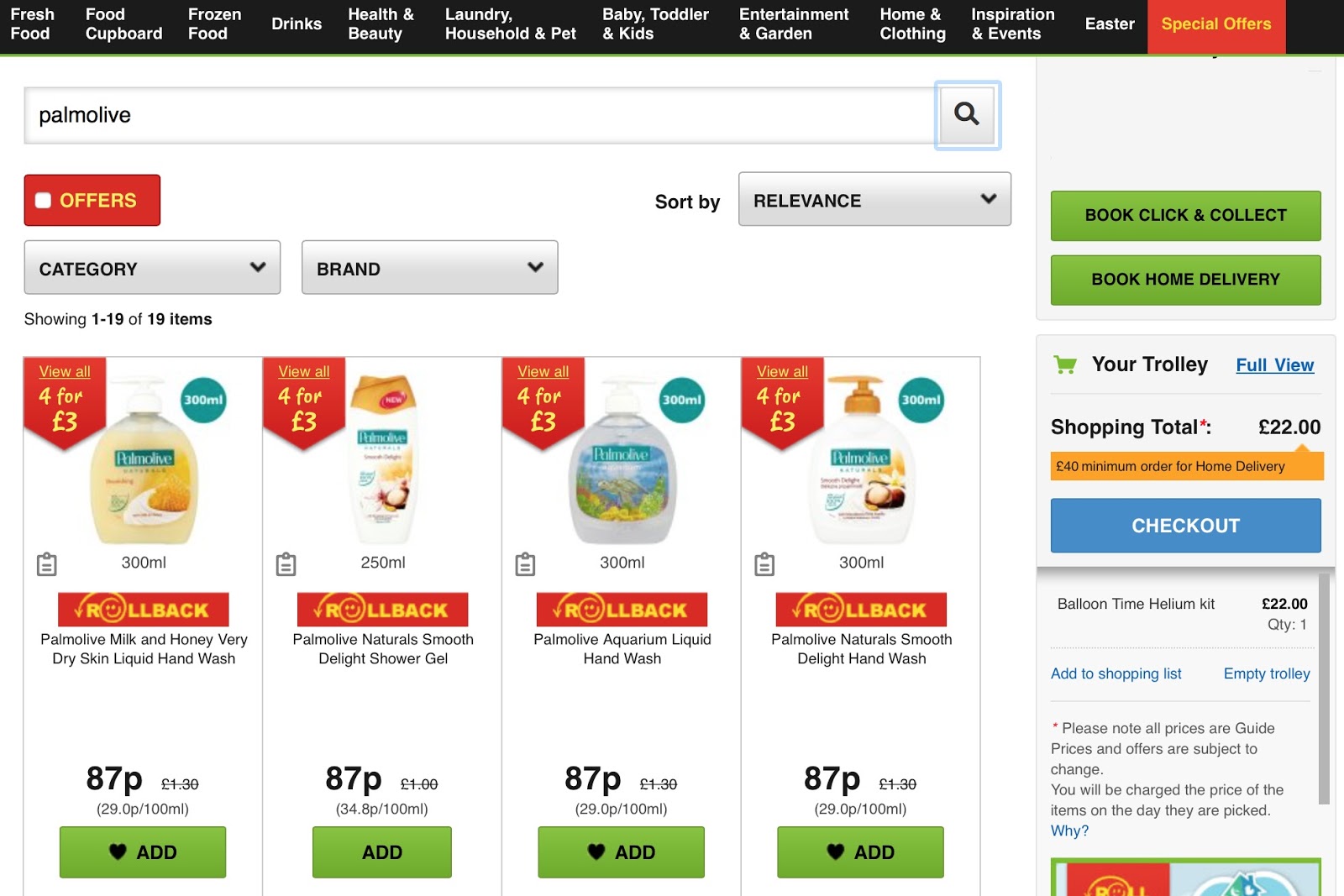This detailed caption describes an online grocery store website interface:

"The image depicts an online grocery store website. At the very top, there is a black strip containing various shopping categories written in white text. From left to right, the categories listed are: Fresh Food, Food Cupboard, Frozen Food, Drinks, Health & Beauty, Laundry, Household & Pet, Baby, Toddler & Kids, Entertainment & Garden, Home & Clothing, Inspiration & Events, Easter, followed by two notable elements: a yellow rectangle and a red rectangle containing yellow text that reads 'SPECIAL OFFERS.'

Directly under this black banner is a search bar with the text 'palm olive' entered, indicating a search for 'Palmolive' products. Below the search bar, there is another red rectangle featuring a white square, alongside which is the word 'OFFICE' written in yellow capital letters.

To the right of these elements is a drop-down menu labeled 'SORT BY,' currently set to 'Relevance.' Below the 'OFFICE' rectangle, there are two more drop-down menus labeled 'Category' and 'Brand,' allowing for further filtering of search results.

The website indicates it is showing items 1 to 19 out of 19 total items. The products listed are all Palmolive brand items, each priced at £4.43. The products include:
1. Palmolive Hand Wash, 300 milliliters, Milk and Honey
2. Palmolive Body Wash Shower Gel
3. Palmolive Aquarium Liquid Hand Wash
4. Palmolive Natural Smooth Delight Hand Wash

Each product entry includes an 'Add to Cart' button below the item’s image. On the far right side of the webpage, there are options for 'Book Click and Collect' or 'Book Home Delivery.' The user currently has a total of £22 worth of items in their shopping trolley, with an option available to check out."